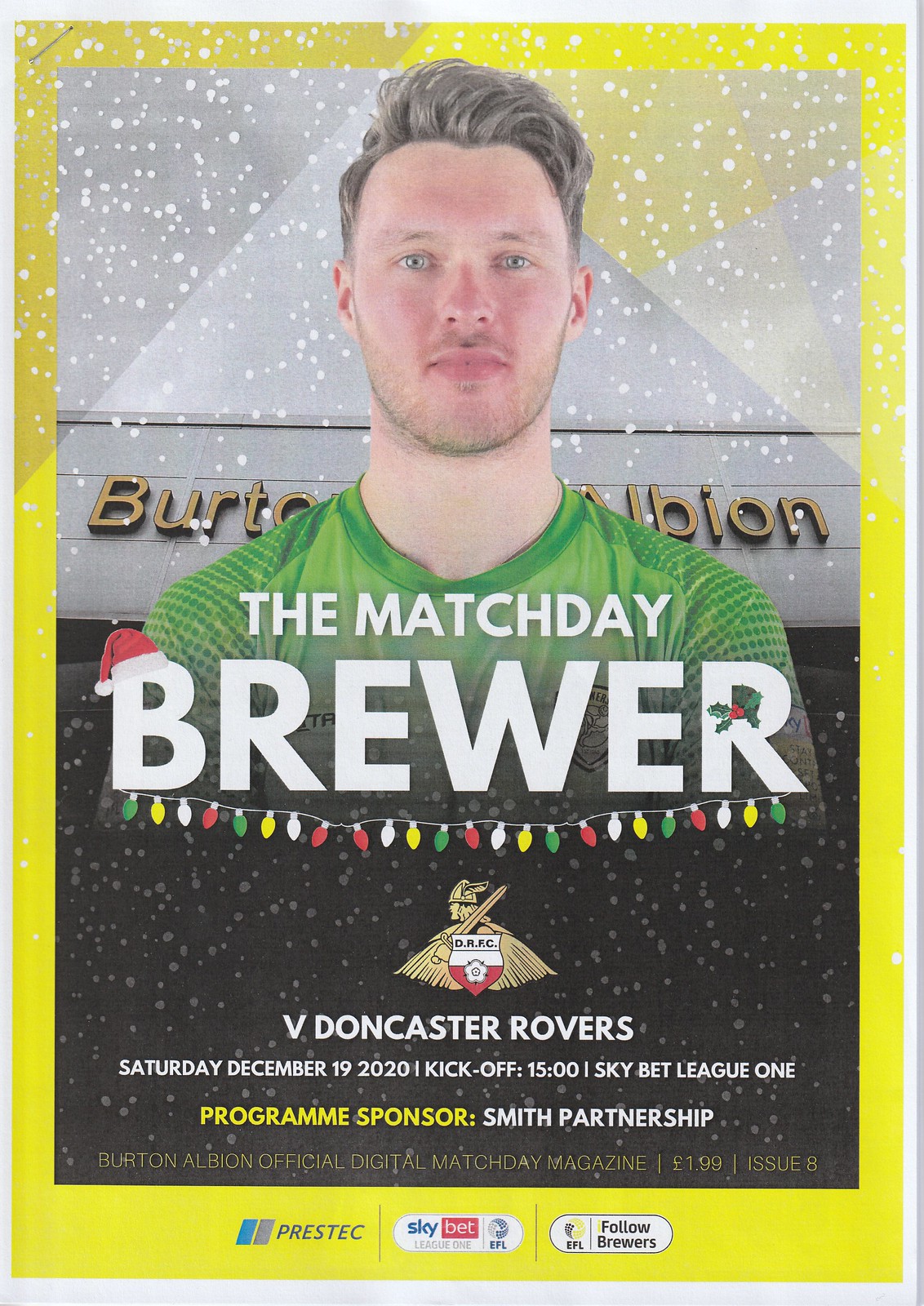The image features a prominently displayed poster with a striking yellow border and a subtle white outline, highlighted by a gray strip along the right edge. At the top left corner, a paperclip secures the poster. Central to the poster is a photograph of a Caucasian man with light blue eyes and light gray hair, which is swooped upwards and slightly to the right. He has a light beard and a subtle smile, and he is dressed in a green jersey, speckled with green details on the shoulders and beneath the collar.

Behind the man's image, partially obscured text reads "B-U-R-T" on the left and "B-I-O-N" on the right. Directly beneath his neck, bold text declares "The Match Day Brewer," with a festive Santa cap perched on the 'B' and a sprig of holly adorning the 'R.' Below this, a string of multicolored Christmas lights—green, yellow, white, and red—adds to the holiday theme.

Continuing down the poster, the emblem of the Doncaster Rovers is prominently displayed: a golden caricature wearing a Viking hat and holding a sword over the shoulder, surrounded by outstretched lines. It features a badge at the bottom that says "D-R-E-C" on a white background, with a red section below.

Text underneath outlines match details: "V. Doncaster Rovers, Saturday, December 19th, 2020, kickoff, 15:00, Skybet League One, Program Sponsor: Smith's Partnership." At the bottom, additional sponsor logos are visible, including Prestix, Skybet, and Follow Brewers. The entire composition exudes a festive and sports-oriented vibe, capturing the essence of an official digital match day magazine, priced at £1.99 for issue 8.